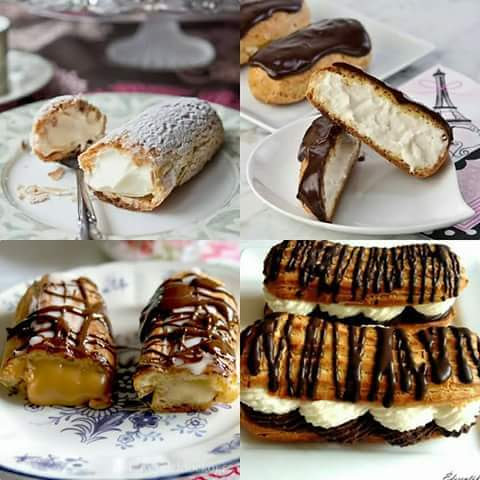The photograph is a vibrant montage split into four equally sized squares arranged in a two-by-two grid, each showcasing delectable profiterole-type desserts on various plates. In the top left image, a profiterole cut in half diagonally at a 7 o'clock angle reveals luscious white cream spilling from its core, with powdered sugar dusted over the golden pastry. This dessert rests on a white plate with a subtle gray floral edge and comes with a stainless steel fork, the handle facing the viewer, while the bottom edge of a crystal cake stand peeks into the frame. The top right image features a complete profiterole bathed in a rich chocolate sauce, elegantly zigzagged across its surface. The pastry sits invitingly on a simple white plate, partly obscured by a napkin illustrated with the Eiffel Tower. In the bottom left corner, another halved pastry, this time filled with a rich cream filling that hints at caramel or a buttery white frosting, is presented on a white plate adorned with a delicate blue floral design, complete with drizzles of chocolate atop. Finally, the tightly cropped bottom right photograph captures two profiteroles layered like sandwiches, filled with a contrasting duo of white and chocolate cream, with the entire scene dominated by a drizzle of chocolate sauce, rendering the plate almost invisible beneath the indulgence.